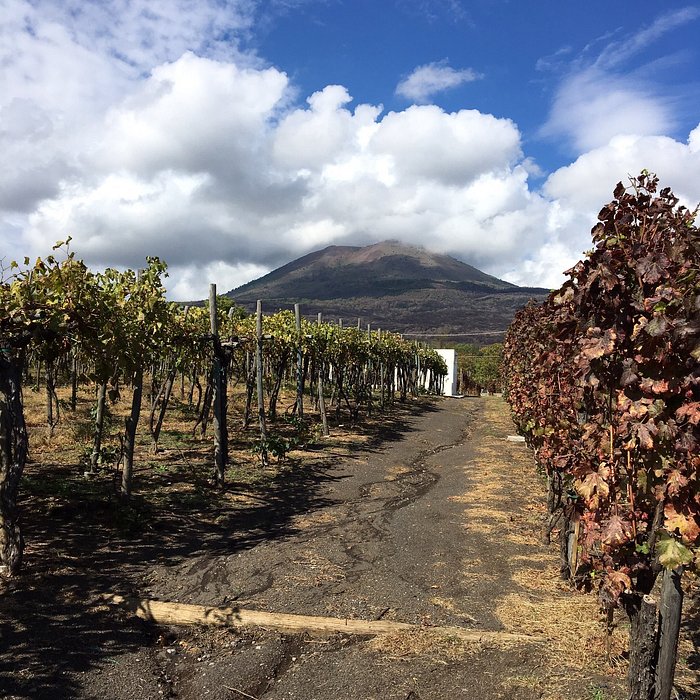This detailed photograph showcases a vibrant vineyard set against a dramatic landscape. In the foreground, starting on the bottom right, a neat line of grapevines emerges, their leaves showing hues of green and red, indicative of the winemaking process. These vines are supported by posts, and further to the left, additional rows of grapevines stretch into the distance, creating an organized and cultivated appearance. Between these rows of vines lies a tan concrete walking path that starts at the bottom of the image and extends towards the center. 

As we move our gaze toward the background, a captivating mountain dominates the scene, possibly a volcano due to its distinct shape, centered perfectly in the frame. This mountain is shrouded by a partly cloudy sky, with patches of light blue peeking through. The colors in the image include the earthy shades of reddish-brown and gray, the lush greens of the vegetation, and the crisp whites of the clouds.

Additional details enhance the scene's complexity: a white rectangular building is visible in the distance, and power lines suggest the presence of a nearby road. This peaceful and scenic setting, captured during the day, embodies the rustic charm of a winery or agricultural farm, reflecting both its beauty and the industrial elements that support it.